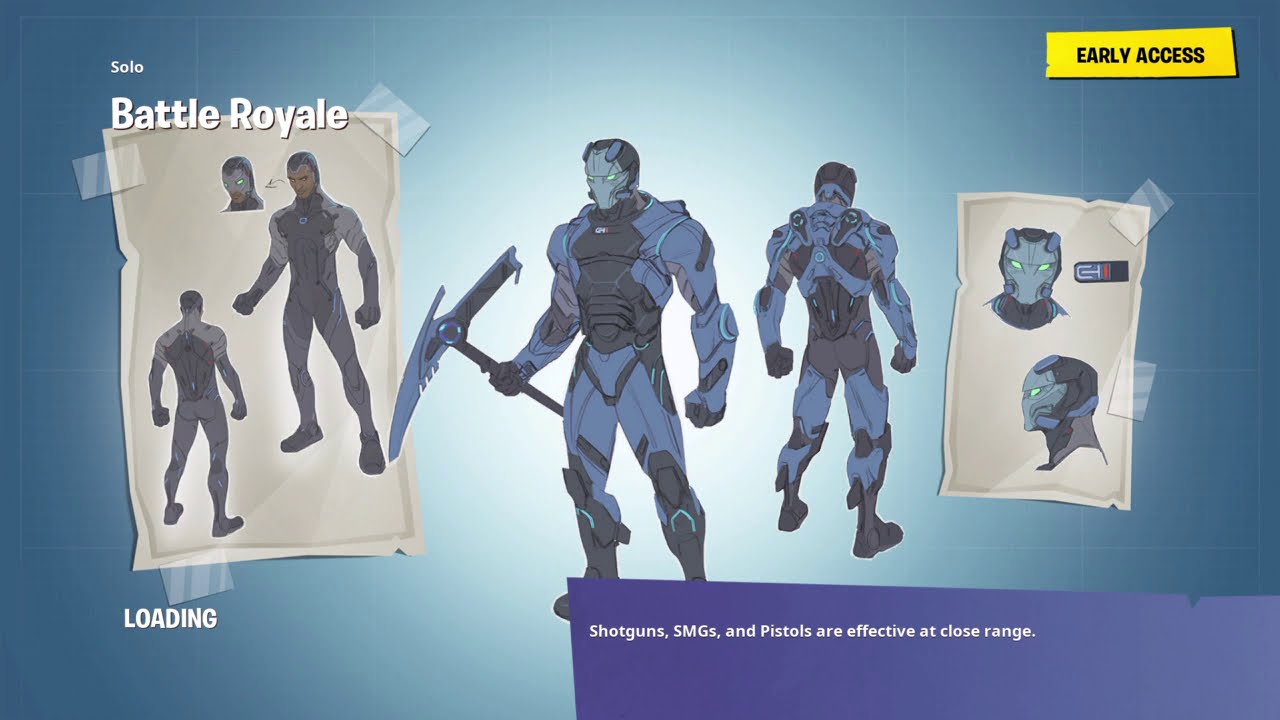The image depicts a screen from a video game with a teal background, highlighted by white lighting in the center. In the upper left-hand corner, it says "Solo Battle Royale" while the lower left-hand corner displays the word "Loading." The upper right-hand corner features "Early Access" in a yellow bar, and the bottom right-hand corner has a message stating, "Shotguns, SMGs, and Pistols are effective at close range."

Central to the image are multiple depictions of a character. Dominating the center are front and back views of a video game character dressed in blue body armor and wielding a sleek, futuristic sickle-like weapon in his right hand. This character has a masked face, adding to the enigmatic appearance. To the right of these images is a representation of a crinkled piece of paper, which appears to be taped to the screen. This paper shows headshots and a profile view of the same character in a helmet. On the left, another piece of seemingly crumpled paper, also taped to the screen, displays images of the same character wearing a spandex costume with less armor, highlighting different perspectives of their design.